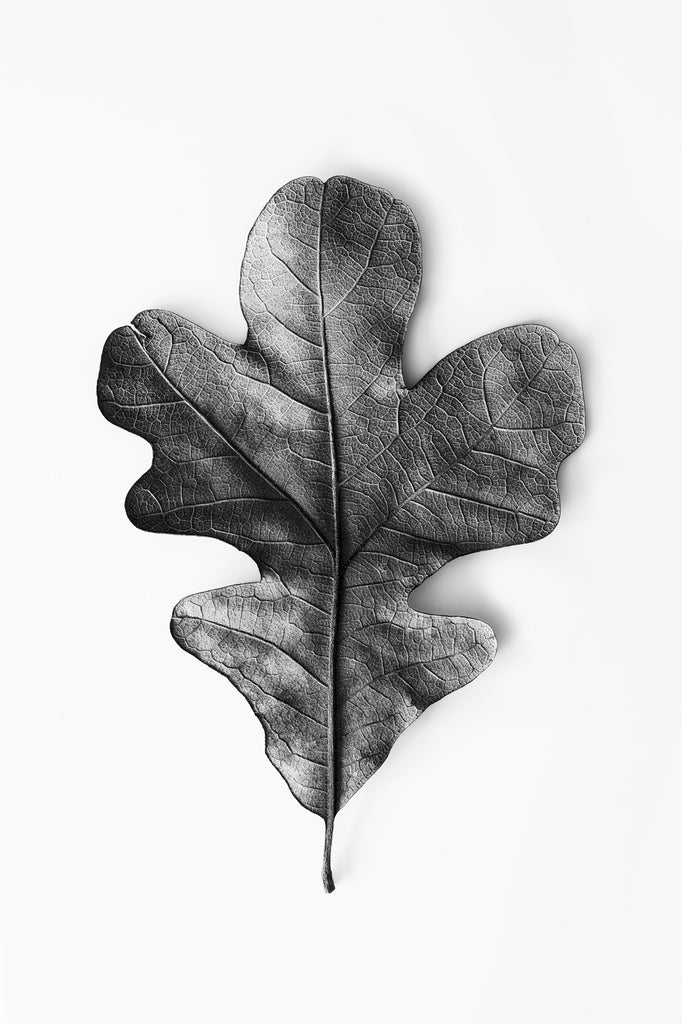The image is a black and white photograph of a tree leaf, displayed against a light grey background. The leaf is depicted in a vertically elongated format, complementary to its naturally tall and narrow shape. Centrally positioned, the leaf dominates the composition with its intricate vein structure. The main veins form a Y-pattern, with one branch extending straight up, and the other two diverging left and right. The leaf showcases five distinct protruding parts: one at the top, two on the upper sides, and two on the lower sides. The delicate veins and wrinkles are meticulously captured, with tiny lines extending throughout the leaf, illustrating its complex biological structure. A small stem at the base of the leaf adds to the detailed rendering, emphasizing the elegance of its form. Despite being in black and white, the photograph captures the rich texture and intricate details of the leaf, making it a striking and contemplative piece.